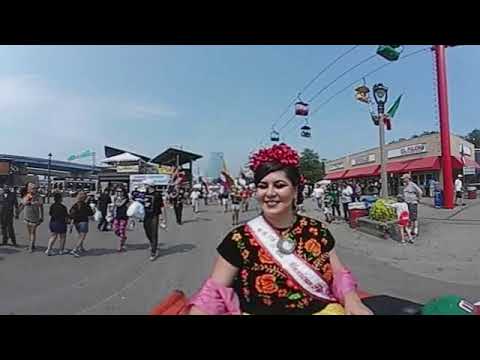In this vibrant street scene, a smiling woman with fair skin stands prominently in the foreground. She wears a black short-sleeve shirt adorned with colorful floral patterns and a white sash with red borders draped diagonally across her chest. On her head, she sports a red floral headdress, adding to her colorful and cheerful appearance. The background reveals a bustling environment, featuring numerous people walking about on a gray asphalt surface, enjoying what appears to be a sunny day with a mostly blue sky and a few hazy clouds. Surrounding the scene, buildings line the street with red awnings, and there's a canopy setup as well as a gondola lift with multicolored cars and a red support pole visible on the right. A distant bridge with street signs adds depth to this dynamic urban or amusement park setting.